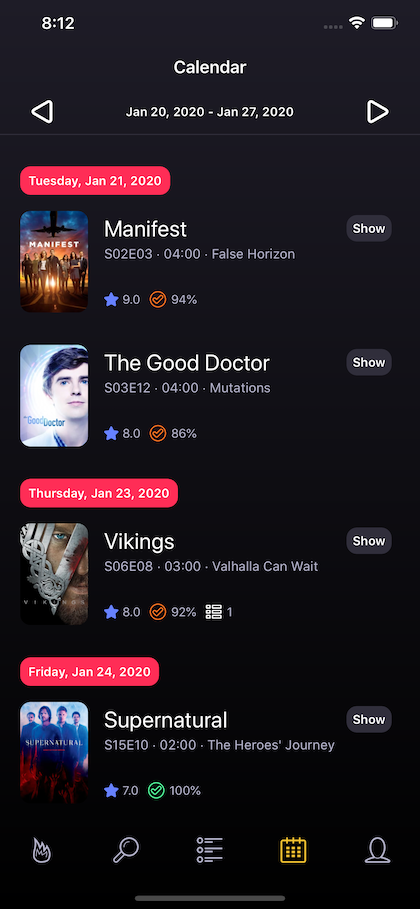The image displays a user interface screen with various details. In the top left corner, there is a small black box showing "8-12" and a nearly full battery icon. Below this section, in the middle of the screen, there is the word "Calendar" followed by the date range "January 20, 2020, to January 27, 2020" accompanied by left and right arrows on either side.

Beneath the calendar section, there is a red box highlighting specific dates and TV show details. One entry states "Tuesday, January 21, 2020," and below it, "Manifest, Season 2, Episode 3 — False Horizon" is displayed along with a star rating of 9.0 and a 94% approval rating. An icon of the cast appears to the left of this information.

Following this, there is another TV show listed: "The Good Doctor, Season 3, Episode 12 — Mutations," with a star rating of 8.0 and an 86% approval rating next to an orange checkmark. An icon of a man with brown hair appears beneath this information. The final red box notes "Thursday, January 23, 2020."